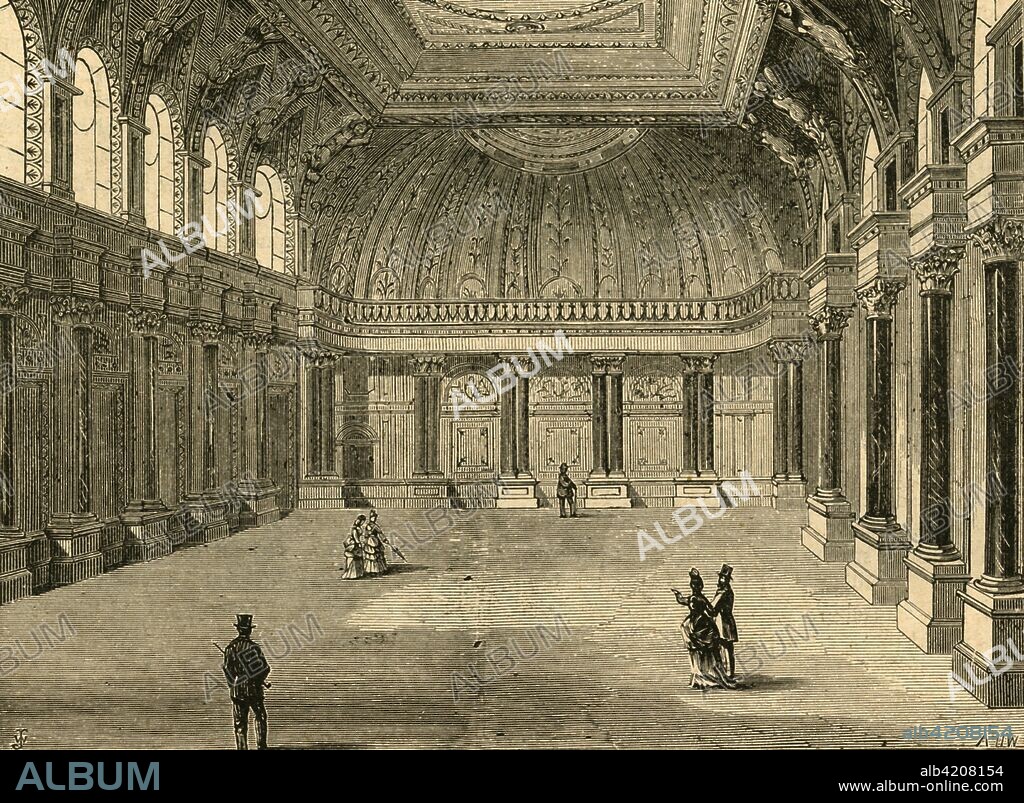The image in question is a meticulously detailed, black-and-white pen and ink sketch of the elegant interior of Draper's Hall. This historic hall features towering ceilings adorned with ornate filigree patterns that curve upward into a tray-like formation. The intricately designed architecture includes numerous vertical columns with square bases and marble finishes, presenting a classical Greek aesthetic. Large arched windows line the top sections of the walls, allowing light to accentuate the room's grandeur. The hall is populated by figures dressed in 1800s Victorian attire, with men in top hats and long coats, and women in elaborate dresses, some carrying walking sticks. The sketch details interactions among the figures, including couples pointing and others strolling or descending what appears to be a staircase. Stamped repeatedly across the image is the word "album," and at the bottom, in green text, is the identifier "ALB 4208154" and the URL "www.album-online.com."